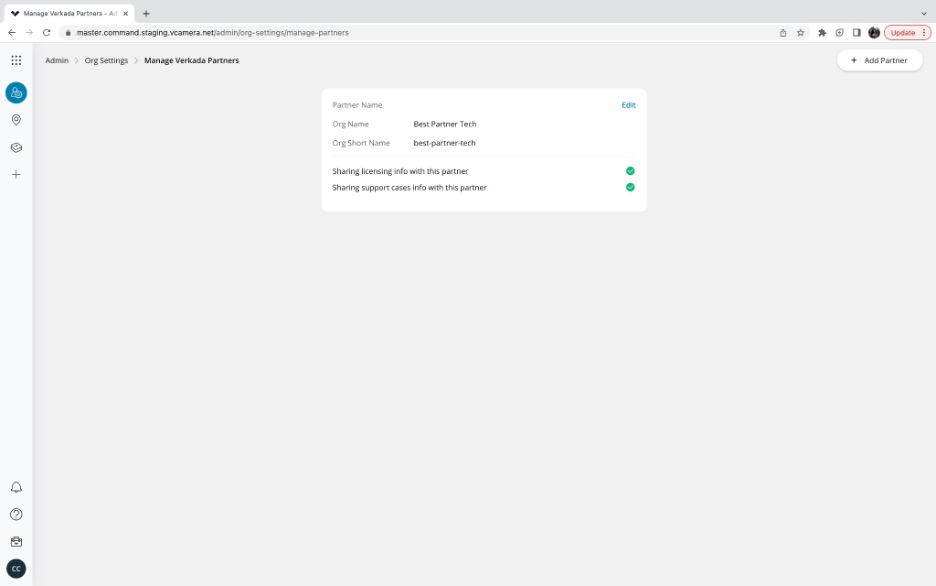Screenshot of a computer interface with a grey theme. The screenshot features a single browser tab open, characterized by its minimalist, grey interface with no visible writing save for a small white pop-up box. On the right side of the screen, there's a vertical navigation bar displaying several options: "Admin", "Original Settings", "Manage", "Vetica Partners", and an option to "Add a Partner." Each of these options is accompanied by green check marks indicating status or completion, except for one marked in red, indicating an issue or incomplete action. At the top, there's a notable header labeled "Update."